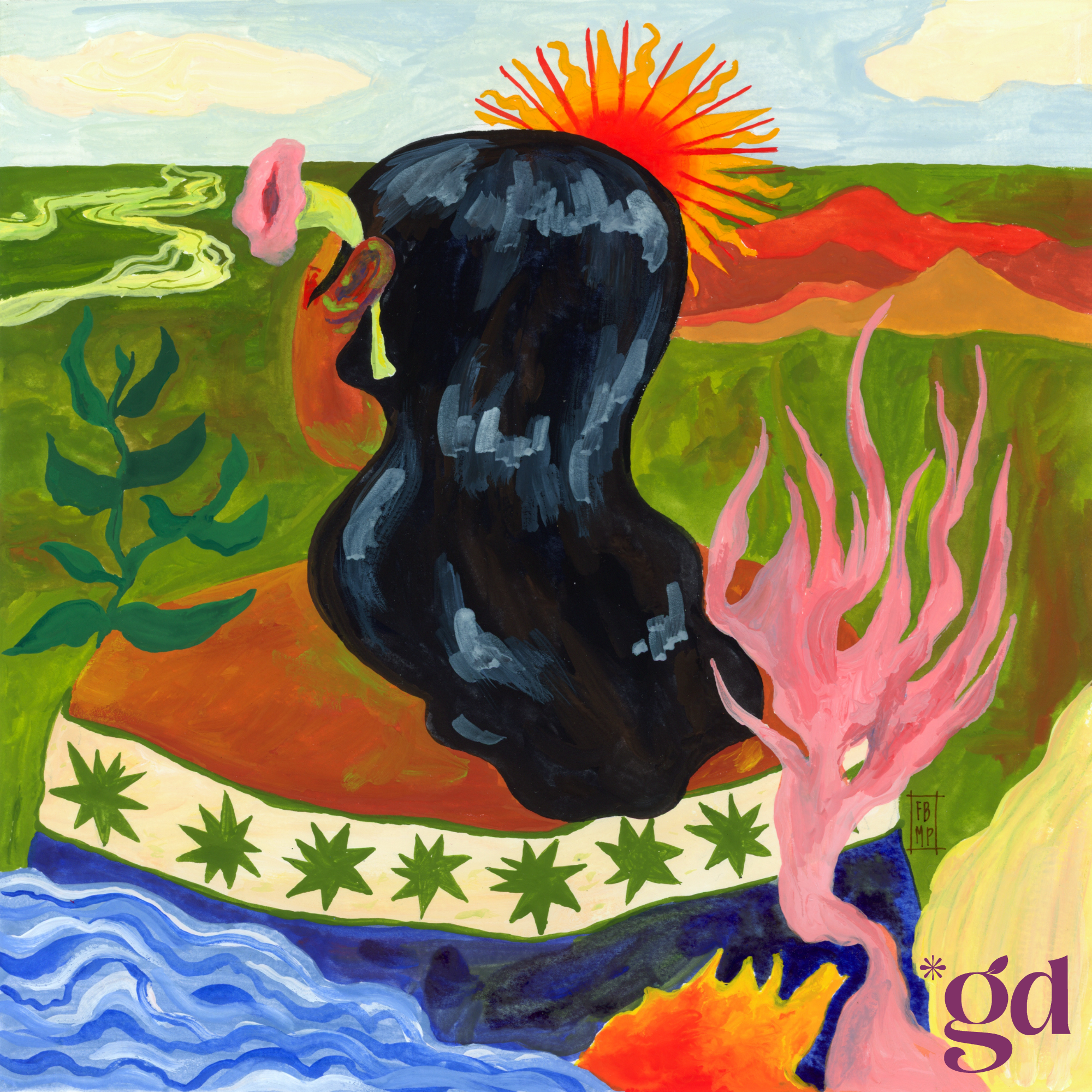The painting depicts a woman with a darker complexion and long, dark black hair that falls to the middle of her back. She has a pink flower with a green stem tucked behind her left ear. The woman, viewed from behind, is wearing a colorful dress adorned with star-like patterns in shades of beige, green, dark blue, and light blue, reminiscent of water. She stands against a vivid landscape, where a radiant sun with orange, red, and goldish-yellow rays dominates the sky, which is a gradient of deep blue with a couple of white clouds.

To her left, a swirling blue stream runs off into the distance, suggesting a watery terrain. Surrounding her are various plants: a prominent pink plant behind her, an orange plant along the bottom, and several leaves or a plant resting on her left shoulder. The background features a broad, expansive green field leading to distant mountain terrain in orange and brown hues. The painting's bottom right corner bears the artist's signature "FBMP" with an asterisk and the letters "GD."